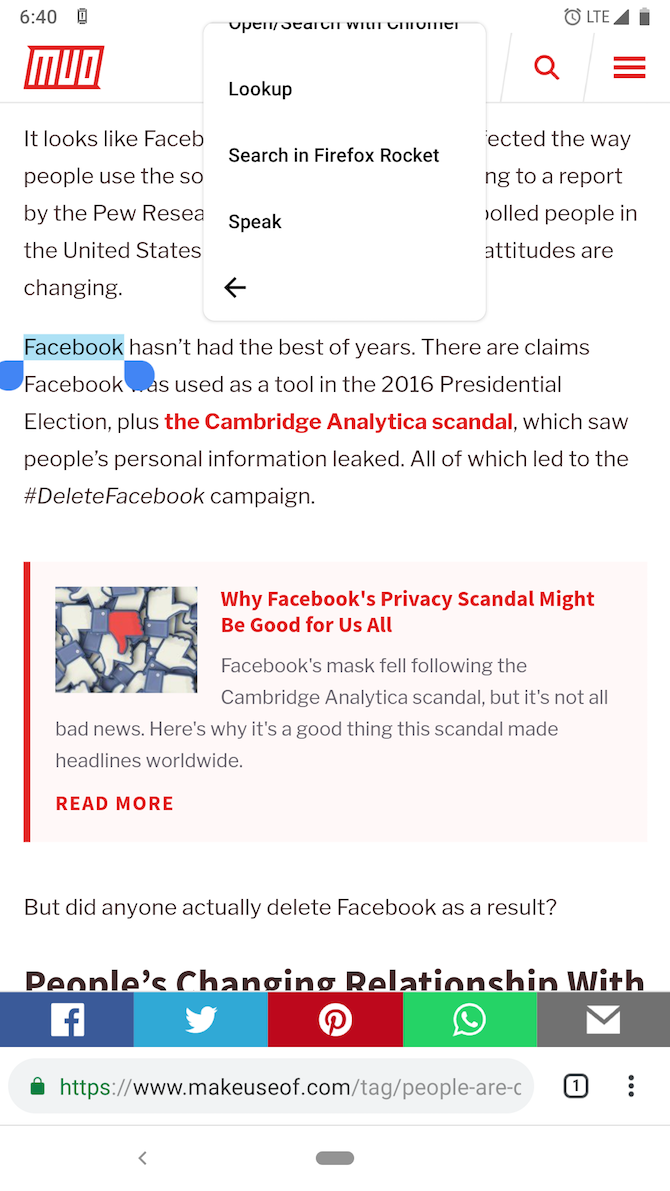This is a detailed screenshot of a website named MUT, identifiable by the logo in the upper left corner featuring white letters with a red outline. In the top section, the time is displayed as 6:40, although it is unclear whether this is AM or PM. A secondary window partially obstructs the main content of the website, displaying the phrases "Look up," "Search in Firefox Rocket," and "Speak," alongside an arrow pointing to the left.

In the visible portion of the website's content, we see a highlighted paragraph beginning with "Facebook," marked in blue. This text reads: "Facebook hasn't had the best of years. There are claims Facebook was used as a tool in the 2016 presidential election plus the Cambridge Analytica scandal, which saw people's personal information leaked, leading to the hashtag delete Facebook campaign." The term "Cambridge Analytica scandal" is emphasized in bold red letters.

Directly below this paragraph, there is a prominent red box featuring multiple Facebook thumbs-up icons. Notably, one icon in the center is red and shows a thumbs-down gesture. The text beside this icon states, "Why Facebook's privacy scandal might be good for us all."